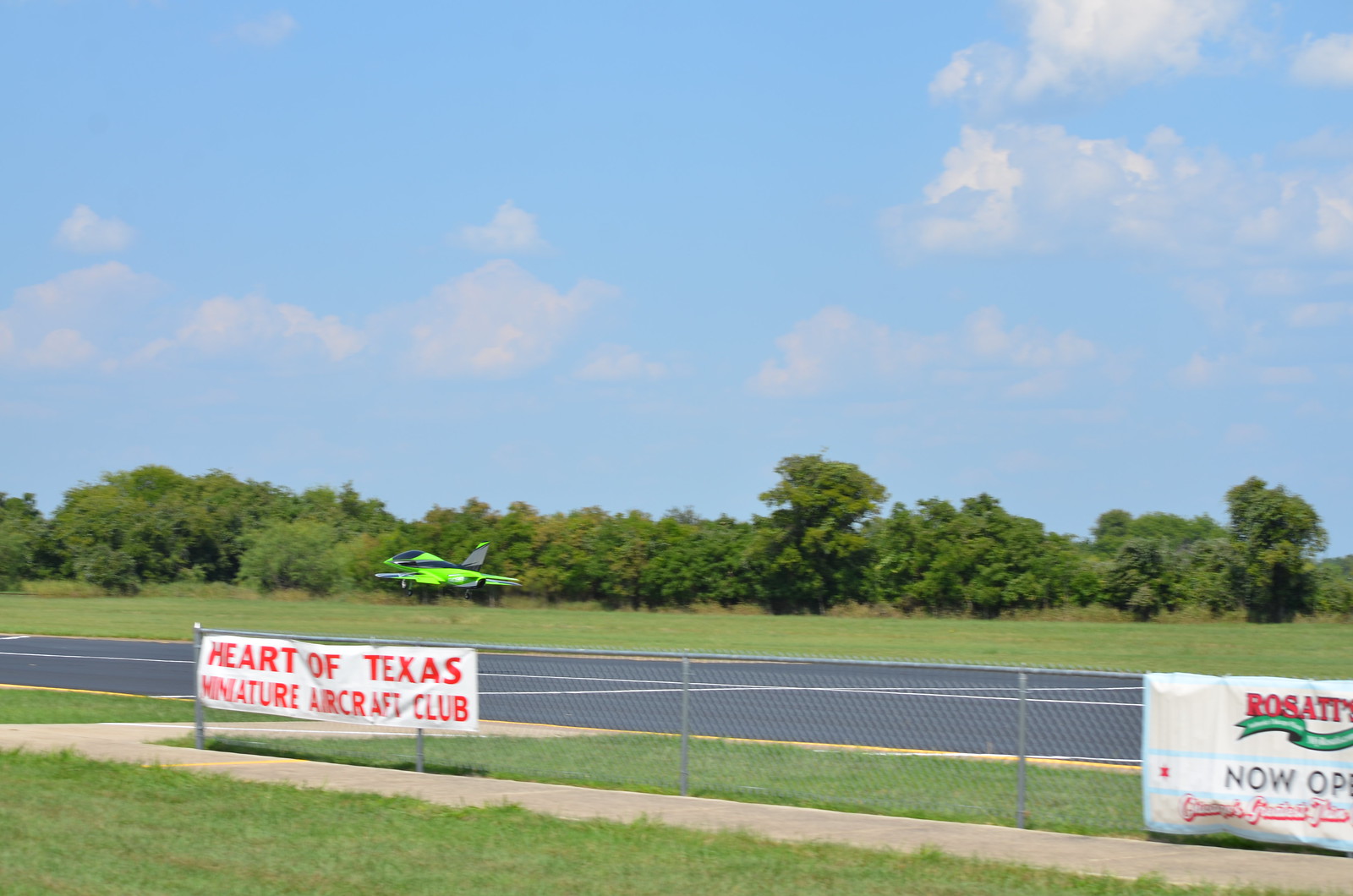In this outdoor daytime photograph, a fluorescent green miniature fighter jet with a distinctive black stripe is prominently featured, parked on a grassy field near a runway. The backdrop reveals a scenic environment with verdant trees under a light blue sky scattered with wispy white clouds. Adjacent to the field is a runway, bordered by grass and lined with clearly painted markings, where a chain-link fence runs along its edge. Attached to this fence are two banners: one reads "Heart of Texas Miniature Aircraft Club" in bold red lettering on a white background, and the other in the bottom right corner announces "Rosati's, now open." The foreground includes a well-maintained grassy area, adding to the overall tranquil yet dynamic setting of this miniature aircraft display.